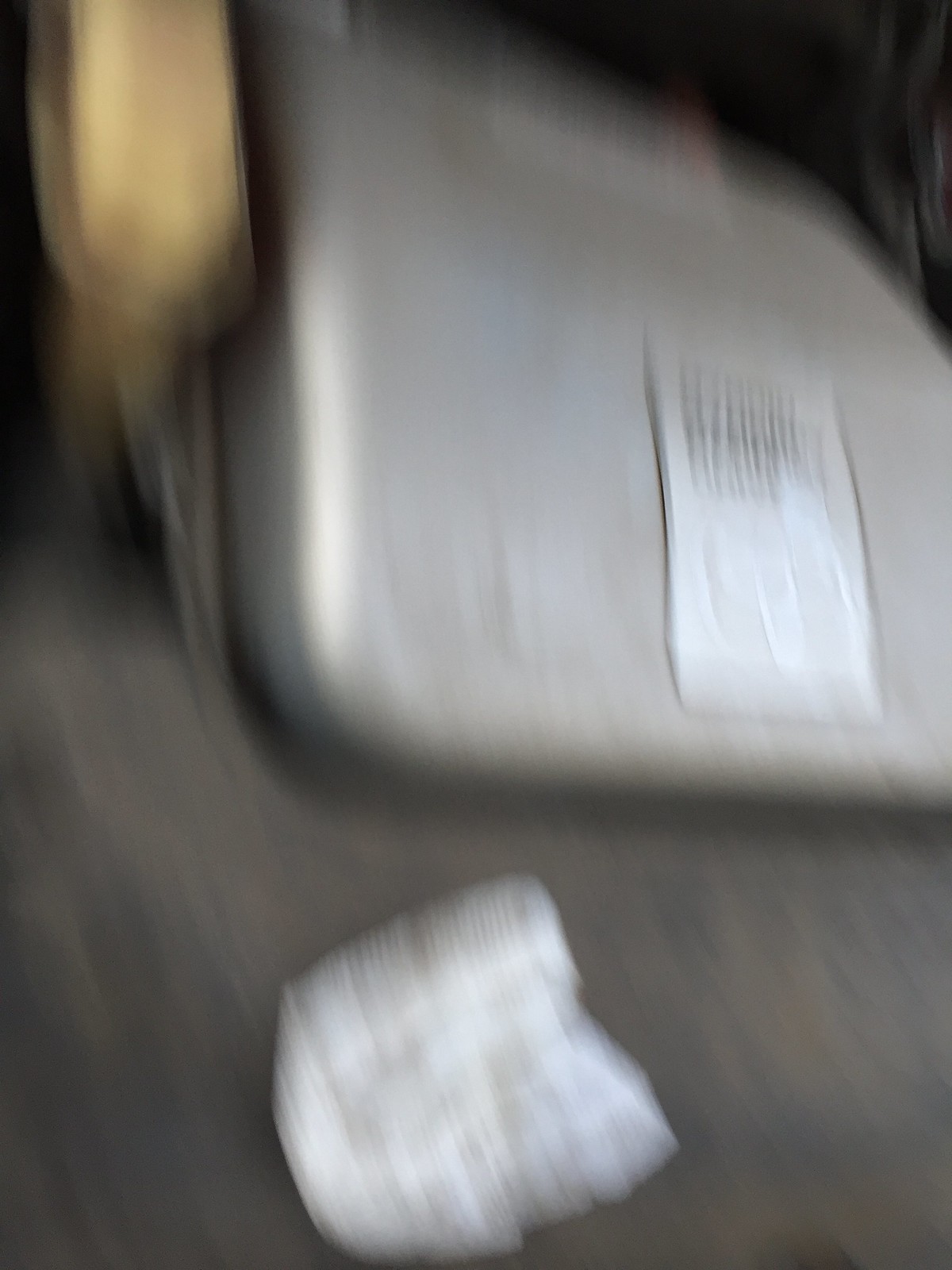A blurry image featuring various objects, including a fabric or plastic seed with a label partially visible underneath. To the left of the seed, there seem to be yellow hues, transitioning to silver on the right side of the seed. The image is out of focus, making detailed identification challenging. The background includes a gray carpeted floor, and a white paper with some text lies on the ground. The photograph also captures a hand in the left portion of the frame and presents noticeable shadows primarily concentrated at the top.